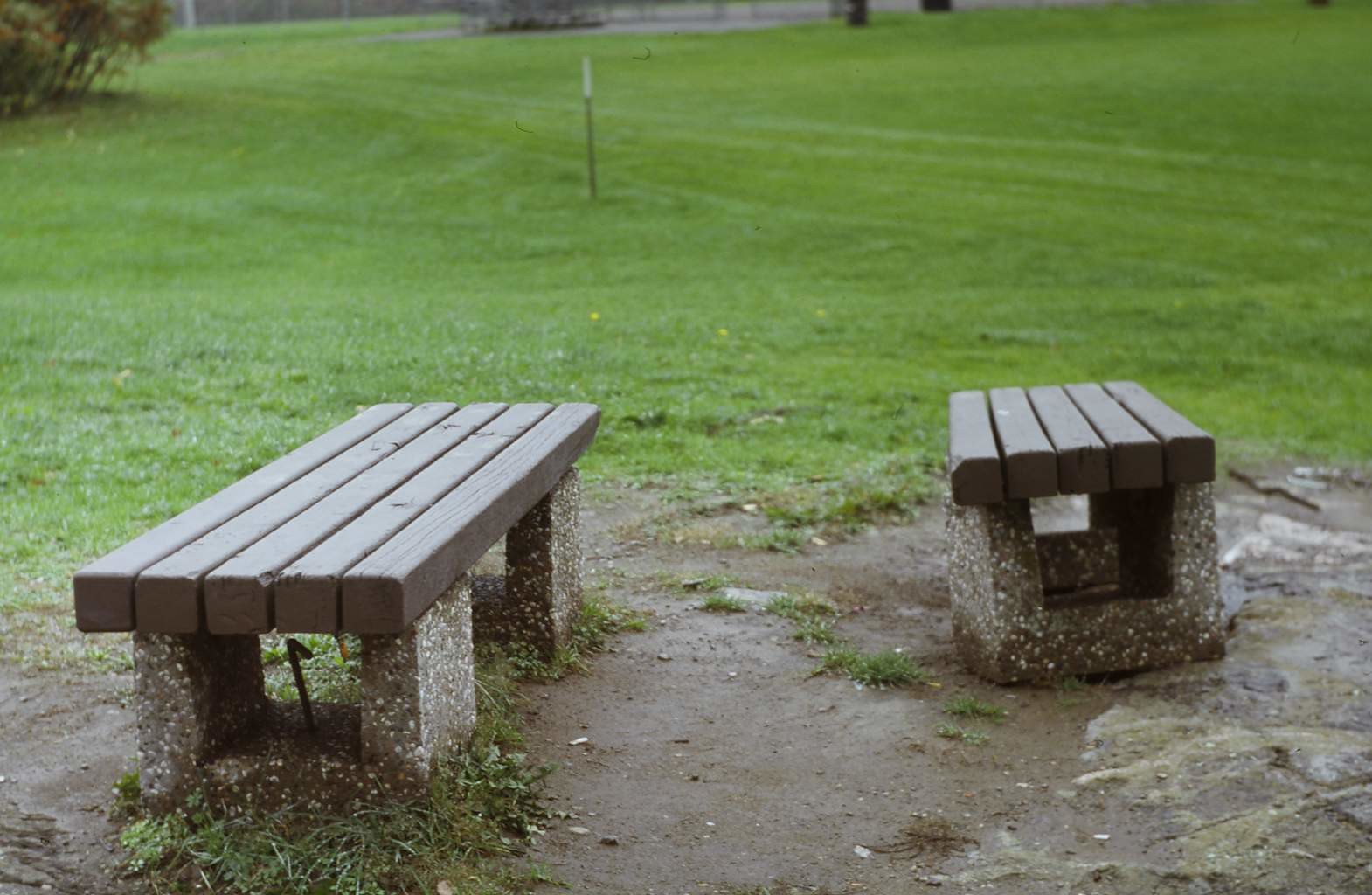The image is an outdoor color photograph taken on a cloudy or overcast day, showcasing two wooden park benches as the central subjects in the foreground. Both benches are crafted with five horizontal wooden beams forming the seat, which rest on rectangular stone blocks approximately five inches tall. The bench on the left is depicted in a three-quarter view with its edge angled towards the viewer, while the bench on the right, though similar in construction, is positioned slightly further back in the same orientation.

The ground immediately around the benches is a muddy patch, likely worn away by frequent use, revealing patches of smooth dirt, small rocks, and some soft mud. This area contrasts with the background, where a large expanse of well-maintained, light green grass stretches out, showing subtle lines possibly formed by foot traffic. In the upper left corner, part of a tree can be seen, and in the center of the upper background, there appears to be a pole. The park seems deserted, adding a sense of solitude to the scene. No text or print is visible in the image.